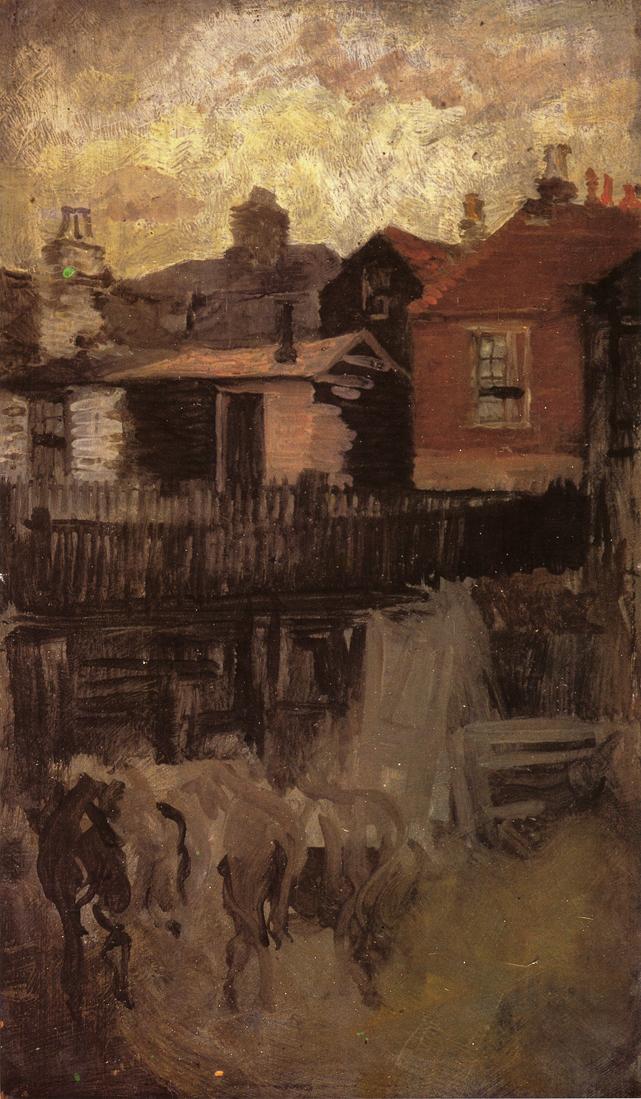This vertical rectangular hand-painted artwork depicts a rustic outdoor scene. The top part features a multi-toned sky blending darker brown with white, transitioning to lighter browns and hints of pink and yellow in a swirly pattern. Below the sky, there is an array of older-looking, wooden houses lined up from left to right: the leftmost houses are light and dark brown, the middle house is dark brown with a red roof, and the rightmost house is red with a brown base. Stretching across the middle of the painting in front of the houses is a brown wooden slat fence. The bottom part of the scene contains abstract, squiggly shapes that resemble horses or cattle in a barn area, with their tails, hindquarters, and heads perceptible yet not sharply detailed. Hints of yellow can be seen in the lower right section, adding to the earthy, rustic palette of whites, browns, reds, oranges, greens, tans, and yellows.